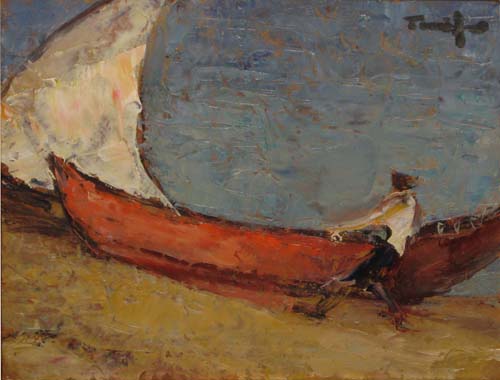The oil painting depicts a picturesque scene of a man pulling a faded red sailboat with a white sail out of the water and onto a sandy shore. The man is wearing a white sleeveless shirt, black pants, and leather boots, and possibly a cap. The sandy beach below is painted in hues of tan, yellow, and orange, providing a stark contrast to the blue water, which is interspersed with specks of gold, brown, and darker blue, creating a wavy, rippling effect. The sail is slightly tilted, giving the impression of movement. The sky or water in the background shares a blue palette, adding depth and emotion to the scene. Brushstrokes are smudgy and expressive, contributing to the painting's emotional and aesthetically pleasing quality. The artist has signed their name in black paint at the top right corner, although the signature is not entirely legible.